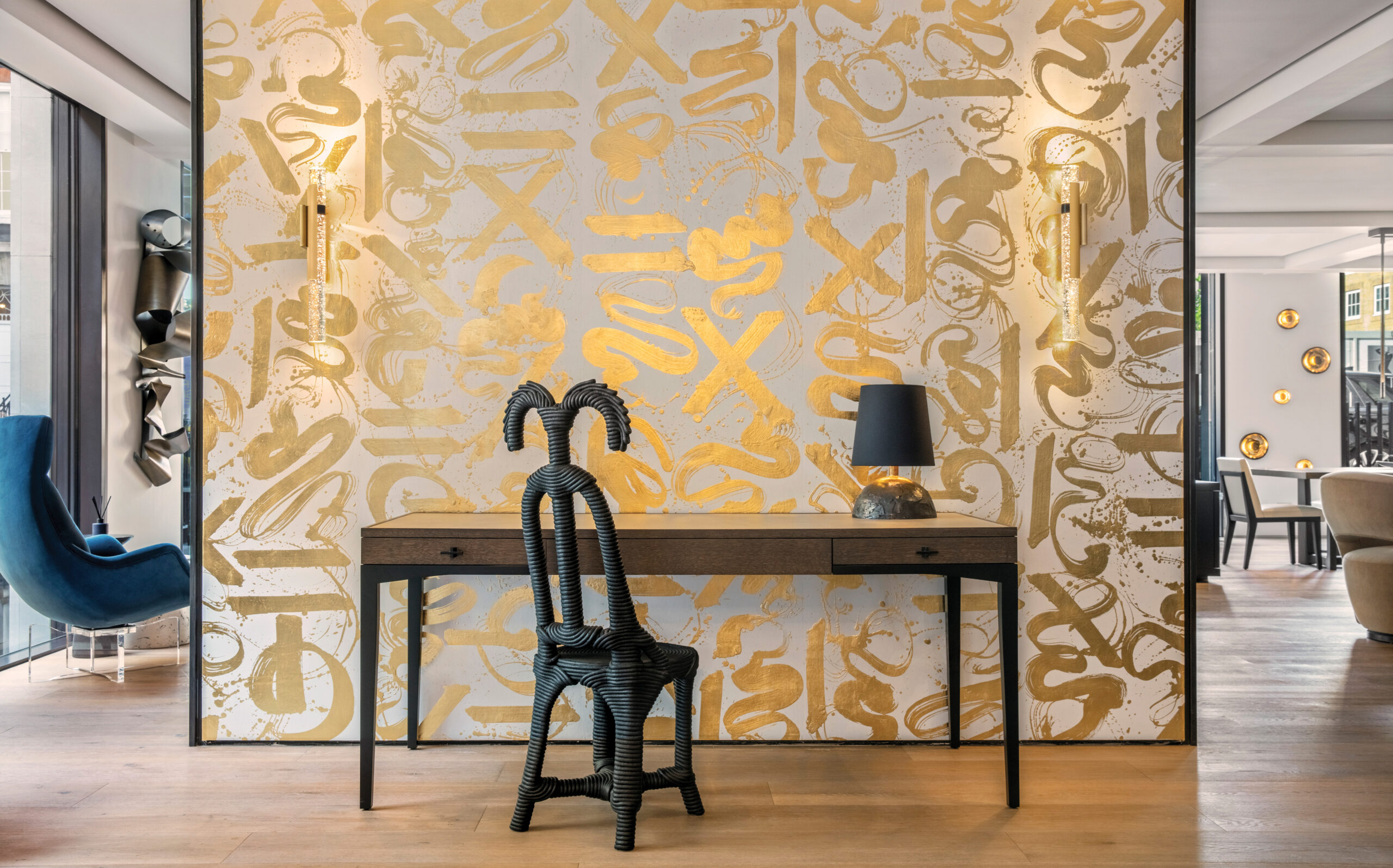The image captures a modern and artistic interior of a home, featuring a distinctively designed workspace. Central to the composition is a compact wooden desk with black legs, topped with a small black lamp with a dark lampshade. In front of the desk sits a striking black wicker chair, adorned with two horn-like structures reminiscent of ram horns extending from its rounded back. Behind the desk, a large, translucent wall panel framed in black and inscribed with gold lettering adds a sophisticated touch. The scene is further characterized by light gray or tan walls and hardwood floors, enhancing the room's modern aesthetic. To the right, there is a table and chairs accompanied by golden wall accents. To the left, a plush blue armchair reclines near what appears to be a sliding glass door, contributing to the room's bright and open atmosphere.